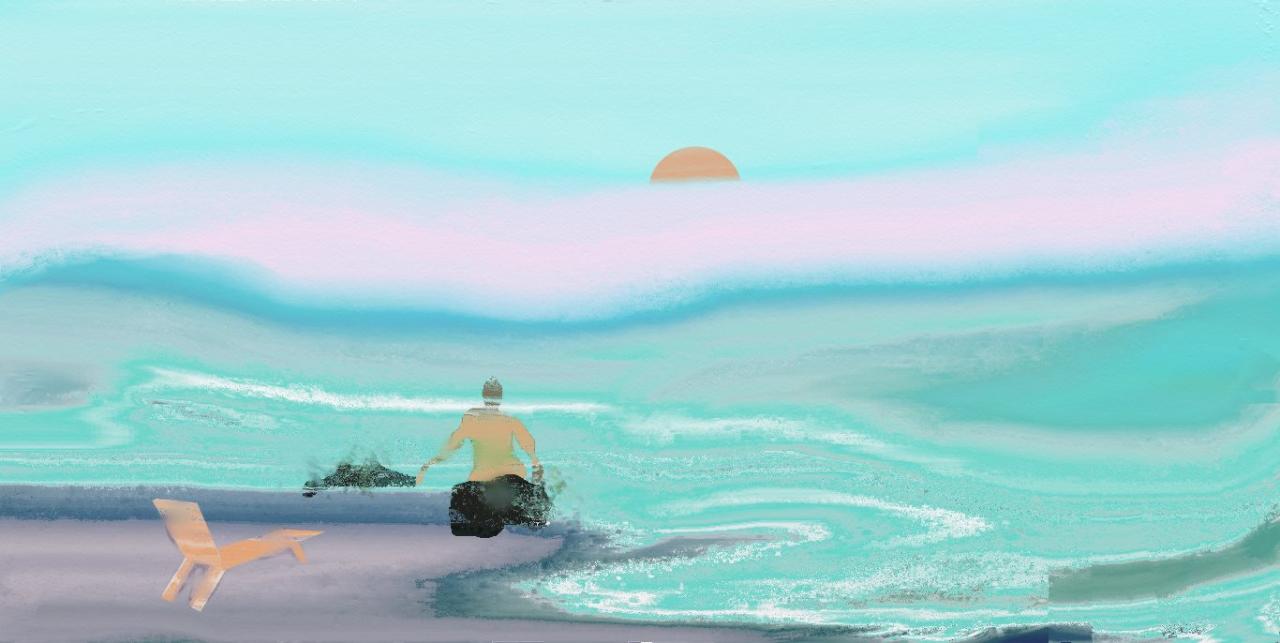"A digitally-rendered image, possibly created using AI, depicts a beach scene with a surreal and slightly amateur aesthetic. The blue ground suggests a sandy shore, though rendered in an unnatural hue. An orange beach chair is positioned on this atypical ground. Swirling patterns of aqua and white mimic the motion of waves coming ashore, albeit with an abstract, somewhat disjointed look. Above, a row of white clouds stretches across the sky, beneath which a half-circle sun peeks out, contributing to the dreamlike quality of the scene. The central figure, viewed from the back, is a human torso, adding an enigmatic human element to the otherwise surreal beach landscape."